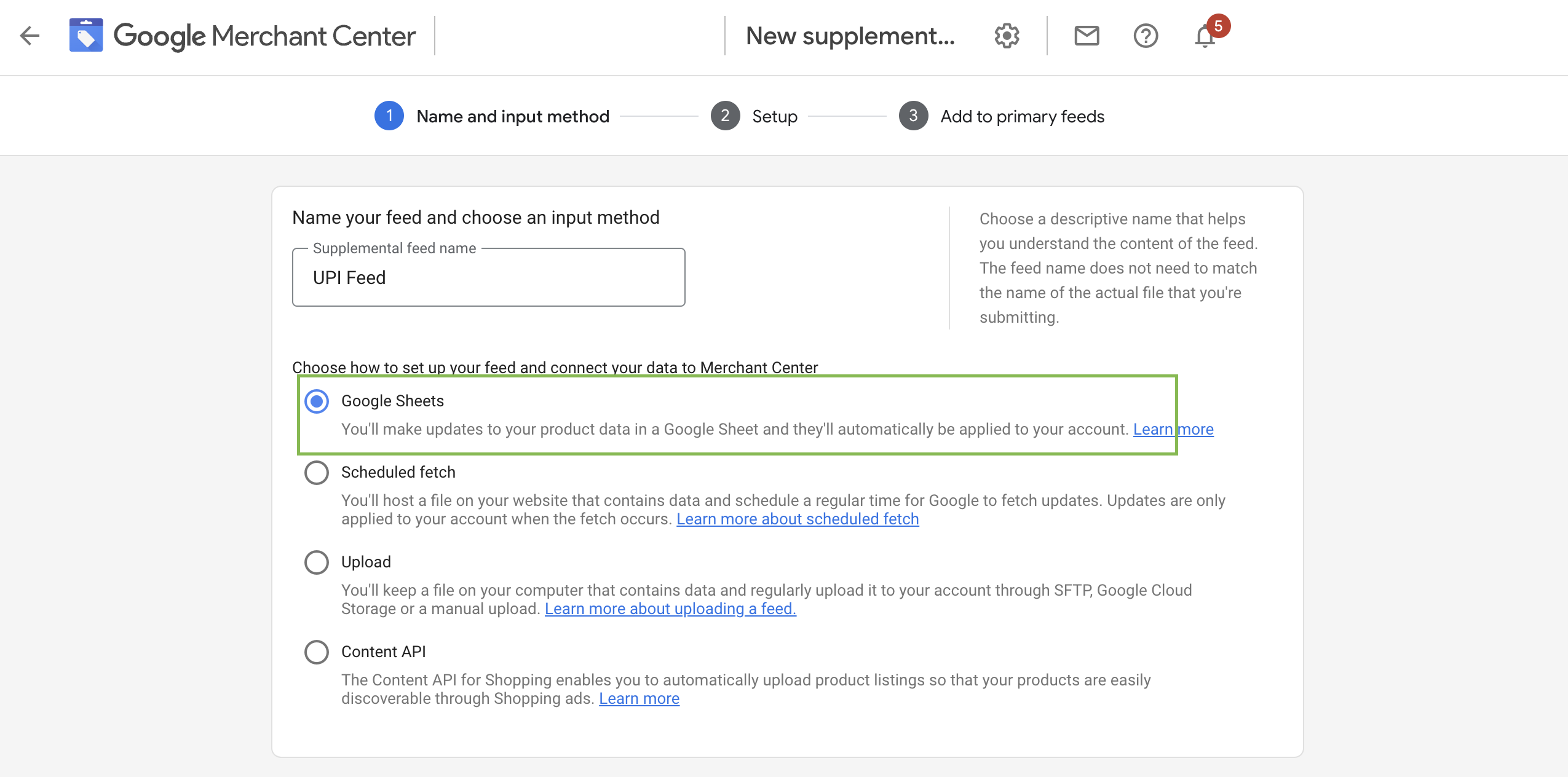The top section of the image displays the "Google Merchant Center" labeled prominently. To the right, several icons are present: a "New Supplement" button, a "Settings Gear" icon, an "Email" symbol, a "Question Mark" for help, and a "Notification Bell" indicating five notifications.

The main section shows a step-by-step guide titled "Name Your Feed and Choose an Input Method." The current supplemental feed name is "UPI feed." Below this, there's advice to choose a descriptive name that helps you understand the content of the feed, noting that the feed name does not need to match the actual file name that you are submitting.

The section continues with a prompt to choose how to set up your feed and connect your data to the Merchant Center. The "Google Sheets" option is selected, with a description indicating that you will make updates to your product data in a Google Sheet, and these updates will automatically be applied to your account.

Below this, three additional options are listed but not highlighted:

1. **Scheduled Fetch**: This option allows you to host a file on your website that contains data and schedule a regular time for Google to fetch updates. Updates are only applied to your account when the fetch occurs.

2. **Upload**: This method involves keeping a file on your computer that contains the data, which you regularly upload to your account through SFTP, Google Cloud Storage, or a manual upload.

3. **Content API**: The Content API for Shopping allows you to automatically upload product listings so that your products are easily discoverable through shopping ads. A "Learn More" link is provided for further details.

The image clearly provides a comprehensive overview of how to name and manage your product feed in the Google Merchant Center, alongside various methods to input and update your product data.